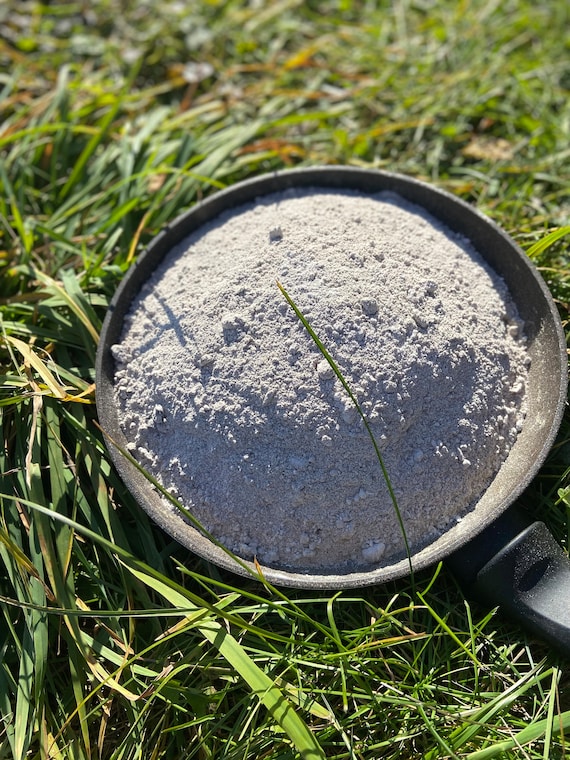The vertically aligned, rectangular outdoor image captured in daylight, showcases a weathered, gray metal bucket filled with a fine, light gray powder, resembling white clay or crushed gravel. The bucket, situated slightly right of center, is surrounded by a ground thick with tall blades of grass, varying from vibrant green to hints of brown, particularly at the bottom where the grass is in clearer focus. As one looks towards the top of the image, the scene blurs slightly. The grass blades are both thin and thick, partially laid down, emphasizing the natural outdoor setting. On the lower right side of the image, there’s a black plastic handle, partially cut off by the frame, suggesting it is unattached to the bucket. Sunlight is shining from the north, illuminating the entire scene.